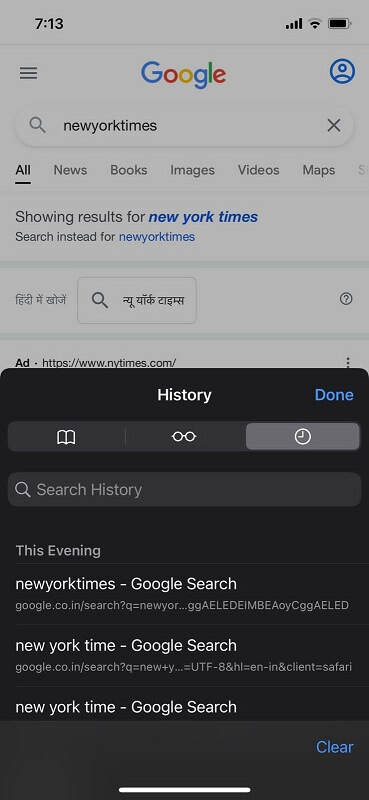This image is a screenshot taken on an iPhone displaying the Safari browser. The top half of the screen shows the Google main page, where the user has entered an unbroken string "NEWYORKTIMES" in the search bar. Google's response displays "Showing results for New York Times" with spaces, and further suggests "Search instead for NEWYORKTIMES" as intended by the user. The brightness of the top half is somewhat dimmed due to the swipe-up menu occupying the bottom half of the screen. The swipe-up menu reveals the Safari browser's history section, set against a black background. Within the history section, a search bar titled "Search History" is visible. The recent search history lists three entries: firstly, "New York Times" (one word as queried), followed by "New York Time" (with spaces), and repeated again with the same "New York Time." This detailed screenshot effectively captures the user's search attempts and browser history within Safari on an iPhone.